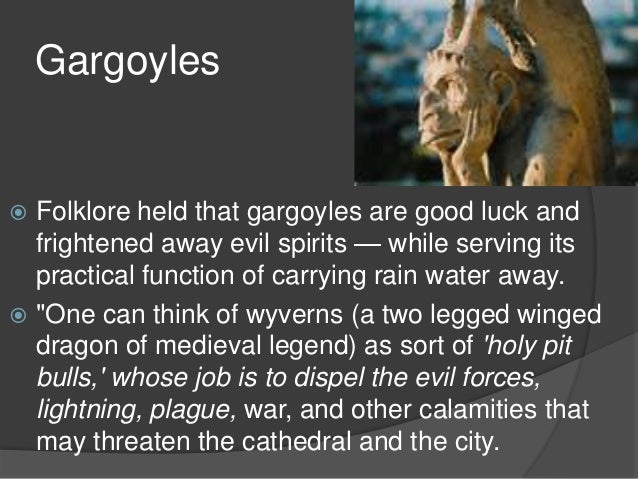The PowerPoint slide titled "Gargoyles," with white text against a dark gray background, features an image of a creamy stone statue of a gargoyle situated in the upper right corner. The gargoyle statue depicts a figure seated with its hands on its face, a pair of horns on its head, elongated nose and mouth, and folded wings extending from its back. The slide contains two bullet points in white text, each accompanied by light blue bullets. The first point reads: "Folklore held that gargoyles are good luck and frightened away evil spirits, while serving its practical function of carrying rainwater away." The second point reads: "One can think of Wyverns, a two-legged winged dragon of medieval legend, as sort of holy pit bulls whose job is to dispel the evil forces, lightning, plague, war, and other calamities that may threaten the cathedral and the city." The overall appearance of the slide is professional and formatted like a typical PowerPoint presentation, featuring a visually distinctive gargoyle statue juxtaposed with descriptive and historical text.